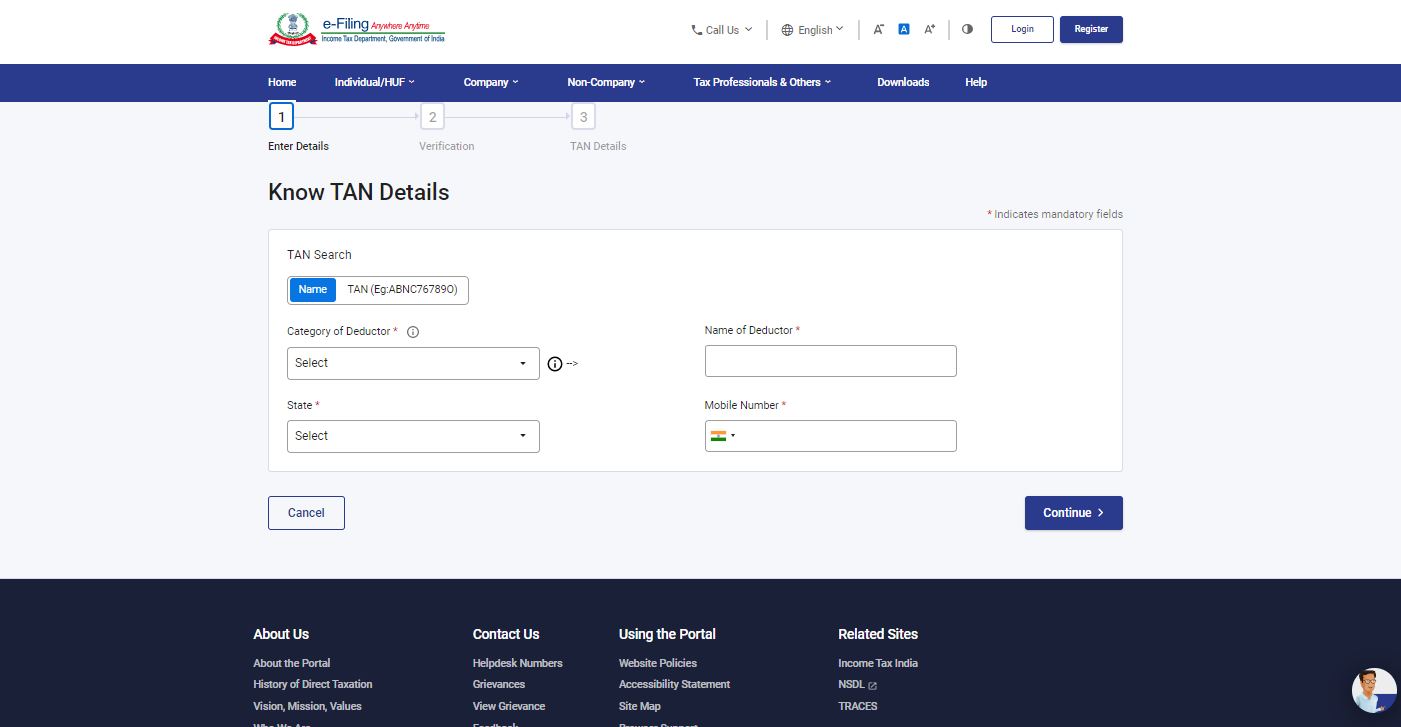This image is a screenshot of a webpage from the Income Tax Department, Government of India's e-filing portal, specifically tailored for accessing TAN (Tax Deduction and Collection Account Number) details. At the top of the screenshot, there is a blue navigation bar with multiple options: Home, Individual/HUF, Company, Non-Company, Tax Professionals, Others, Downloads, and Help. On the right side of the navigation bar, there are additional options for Language Section, Accessibility Settings, and Login/Register buttons.

The title of the page reads "No TAN Details." The page layout is divided into three steps—Enter Details, Verification, and TAN Details—with the current step highlighted as "Enter Details."

The central part of the page features a form titled "TAN Search." This form includes several fields:

1. **TAN**: A text field for entering the TAN number formatted as ABCD67890.
2. **Category of Deductor**: A drop-down menu labeled "Select."
3. **State**: Another drop-down menu also labeled "Select."
4. **Mobile Number**: A text field for entering a mobile number, accompanied by an Indian flag icon indicating the country code.

At the bottom of the form, there are two buttons: "Cancel" and "Continue."

The footer of the page includes links to About Us, Contact Us, Using the Portal, and Related Sites such as Income Tax India, NSDL, and TRACES.

The overall layout is designed to facilitate users in verifying their TAN details for further processing.